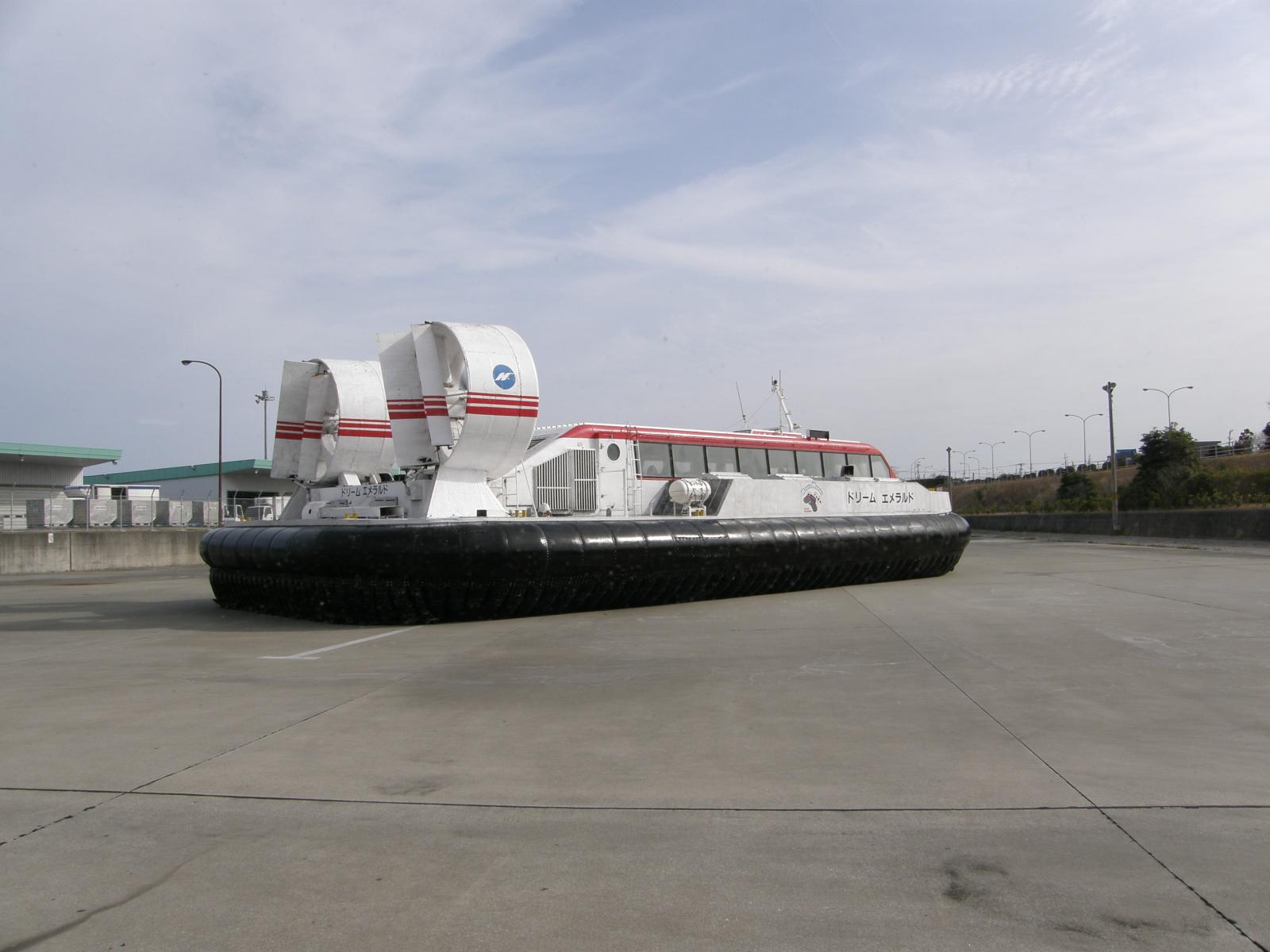This is a photograph of a hovercraft resting on a flat, gray, concrete ground, possibly a parking lot or dock area. The hovercraft's cabin is primarily white with red stripes adorning the upper section, and its underside is clad in thick, shiny, black rubber, giving it a distinct, inflated appearance. The vehicle features two large fans at the back, equipped with directional fins, presumably to aid its hovering and maneuvering capabilities. The cabin is lined with windows and appears to be about one story high, providing space for pilots, crew, and passengers. To the left of the hovercraft, a cluster of buildings and rooms is visible, while the right side shows a grassy area with plants. The sky above is blue and filled with clouds, creating a contrasting backdrop to the scene. Notably, Japanese writing is visible on the side of the hovercraft.